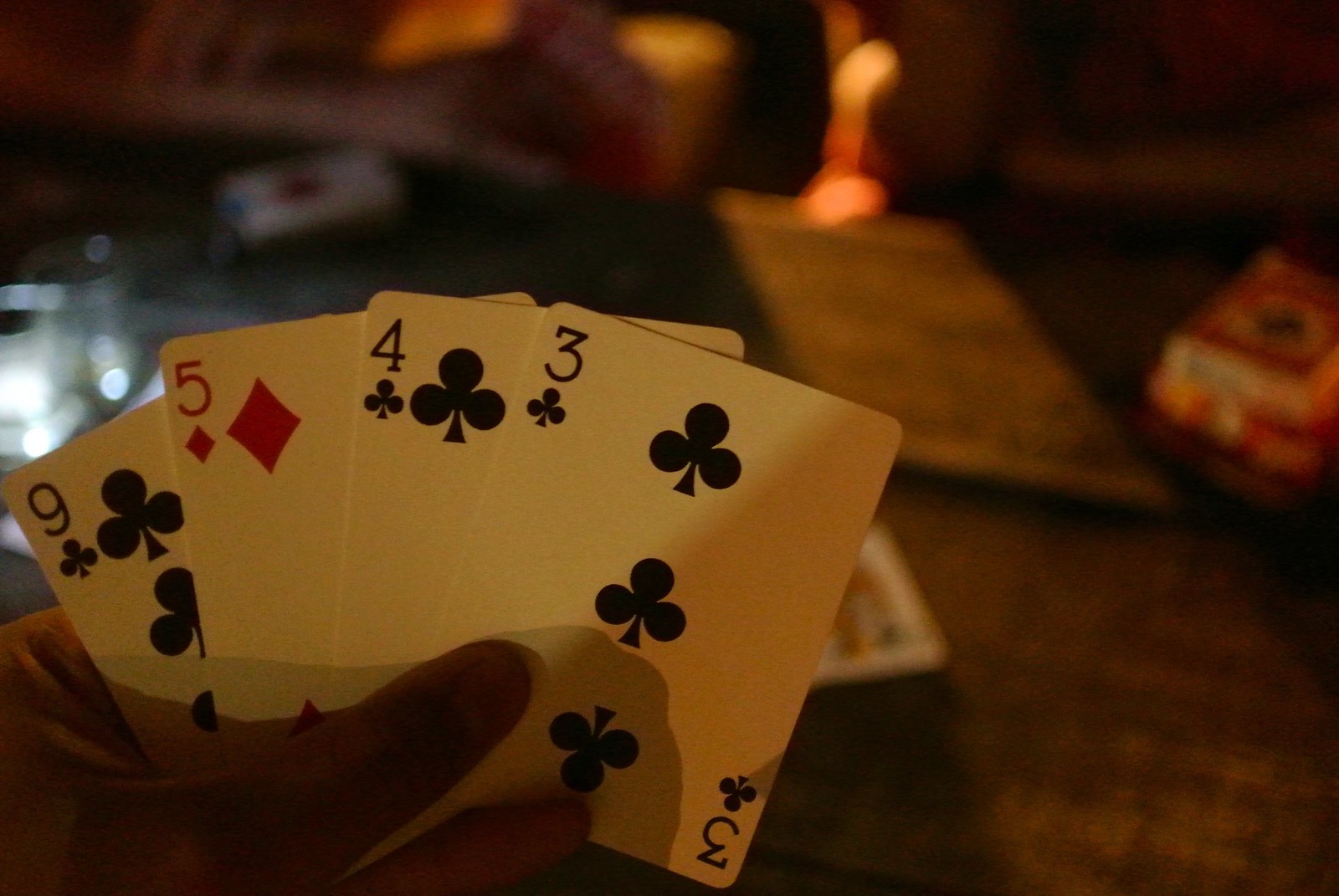In this indoor nighttime photograph taken under poor lighting conditions, a left hand is prominently featured holding a fanned-out hand of playing cards. The cards, identified as a nine of clubs, five of diamonds, four of clubs, and three of clubs, are arranged with the nine at the back. The hand appears to be male. The background is out of focus and mostly dark, but on the right side, a portion of a carpet is visible. The setting suggests the presence of a table, possibly a coffee table or a dining room table with a runner, as some cards are seen lying on its surface. A face card is distinguishable at the bottom right of the table. Behind the cards, on the left edge of the photograph, there is a reflective element, adding a subtle gleam to the scene. At the top of the image, an unidentified pink object is visible, though it is too blurred to discern its nature. The table, if present, appears to be black, further accentuating the dim, intimate ambiance of the photo.